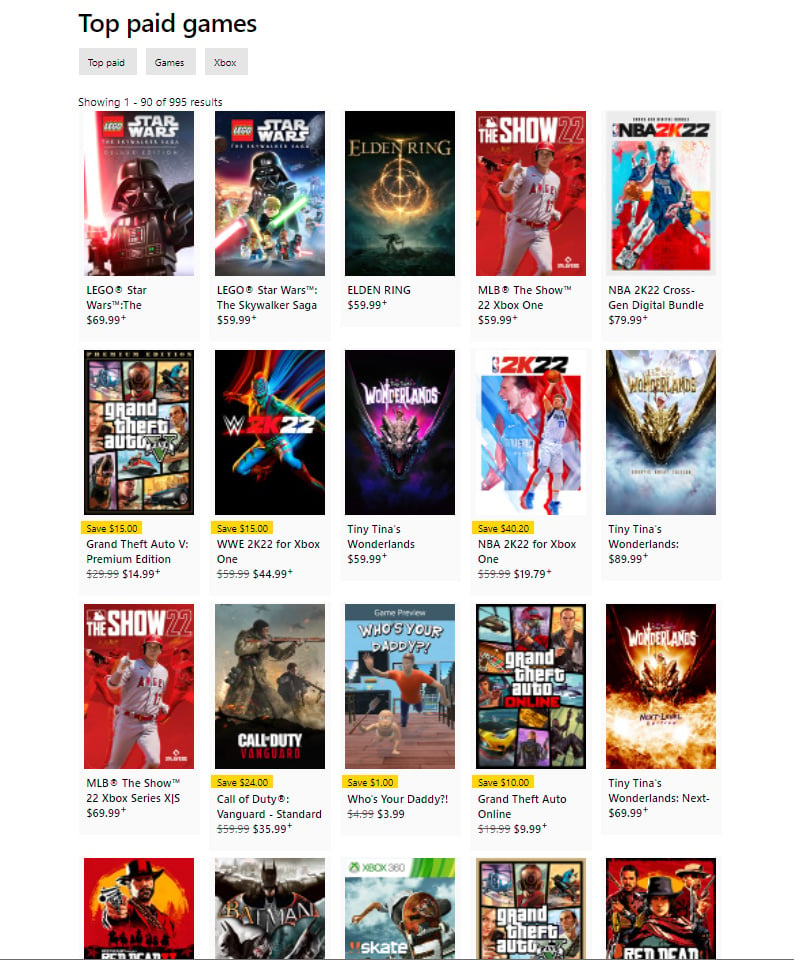A vertical rectangular image titled "Top Paid Games" in black text atop the image. Below the title are three horizontal gray rectangular sections labeled "Top Paid," "Games," and "Xbox" in black font. Just above the list of games, a small black font indicates, "Showing 1 to 90 of 995 results."

The image features four rows, each containing the cover art for five games, with a total of 20 visible games. 

**First Row:**
1. **Lego Star Wars**: The cover prominently displays "Star Wars" in white, slightly right of center. On the left, "Lego" is written vertically in white. The image includes characters resembling Darth Vader and lasers. Below, the text reads "Lego Star Wars" followed by "$69.99."
2. **Lego Star Wars: The Skywalker Saga**: Similar cover art with "The Skywalker Saga" included. Price listed as "$59.99."
3. **Elden Ring**: The cover is darker with a highlighted glow. Priced at "$59.99."
4. **MLB The Show 22**: Features a baseball player in a red cap and gray uniform with red. Text below reads "MLB The Show" on one line, followed by "22 Xbox One" and "$59.99" on subsequent lines.
5. **NBA 2K22**: Displays a basketball player. Text below reads "NBA 2K22 Cross-Gen Digital Bundle" with a price of "$79.99."

**Second Row:**
1. **Grand Theft Auto**
2. **WWE 2K22 for Xbox One**
3. **Wonderlands**
4. **NBA 2K22 for Xbox One**
5. **Wonderlands** (repeated from earlier in the row)

**Third Row:**
1. **MLB The Show 22**
2. **Call of Duty: Vanguard**
3. **Who's Your Daddy**
4. **Grand Theft Auto Online**
5. **Wonderlands**

**Fourth Row (partially visible):**
1. Cut off (partially visible)
2. **Batman**
3. **Skate**
4. **Grand Theft Auto**

Each game cover features corresponding titles and prices in small black font underneath the images. The detailed descriptions and pricing help in identifying and understanding the variety of top-paid games displayed in this particular Xbox listing.